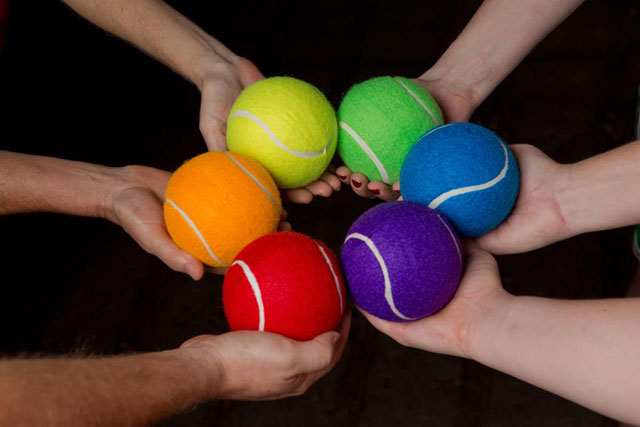In a detailed and professionally arranged color photograph, six outstretched hands and forearms of lighter skin tones form a circular pattern against a completely black background. The hands, extending from various corners and sides of the image, hold large, fuzzy tennis balls in their palms, each ball showcasing a traditional white U-shaped lining. The tennis balls, adding a vibrant splash of color, are arranged in a specific order: starting from the bottom right and moving clockwise, the balls are purple, blue, green, yellow, orange, and red. While most forearms and hands appear smooth, the arm at the bottom left is noticeably hairier. One of the hands features nail polish, hinting at a mix of genders. The composition radiates a floral, sun-like appearance, highlighting the multicolored tennis balls and their unique arrangement.